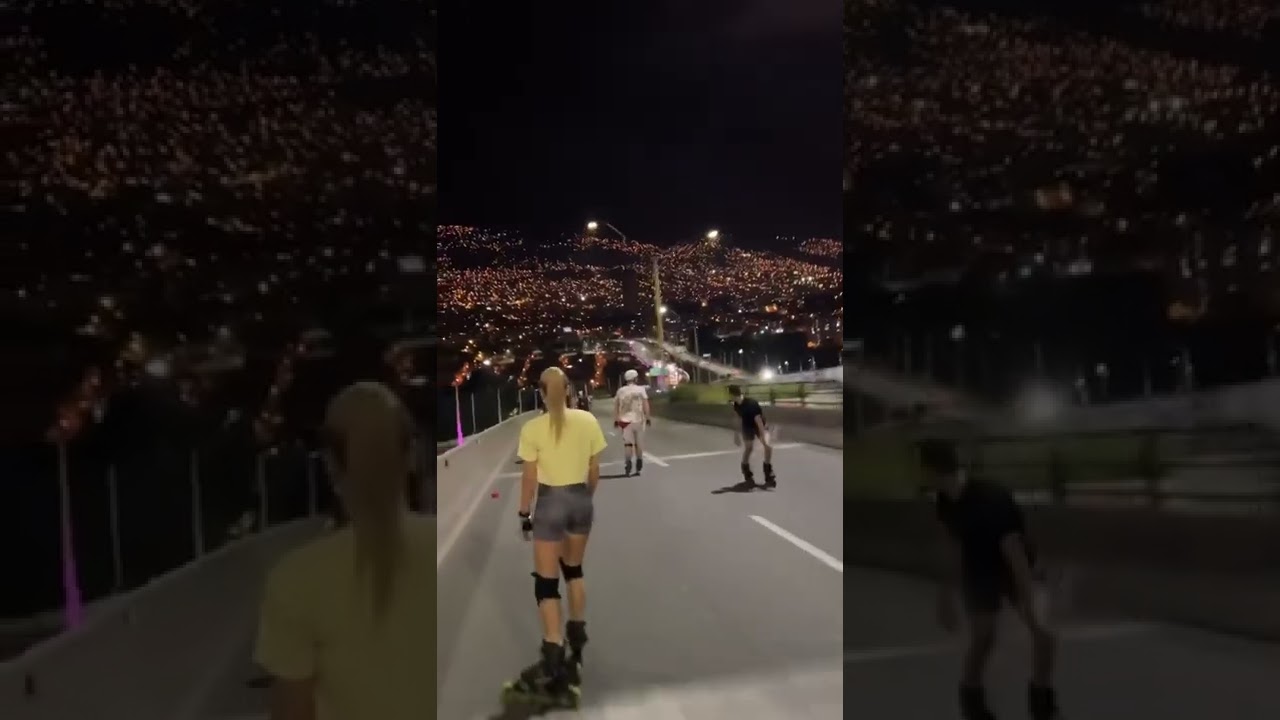This nighttime color photograph, presumably taken on a mobile phone in portrait orientation, appears to be a still image from a GoPro video. To achieve a landscape format, the left and right sides of the original image are filled with a blurred, blown-up repetition of the central picture. The main focus is a group of rollerbladers descending a steep, empty highway. The scene is illuminated by city lights in the distant background, creating a broad and expansive cityscape stretching into the night.

In the foreground, a woman with blonde hair tied in a ponytail is seen from behind. She wears a white shirt, short jean shorts, black knee pads, and black gloves as she glides downhill on her rollerblades. Ahead of her are a few more rollerbladers scattered along the paved road, including one man rolling forward and another dressed in black who is rolling backward, looking back up the hill. The setting is devoid of cars, with large overhead lights casting a stark illumination on the asphalt. The striking contrast between the dark sky and the vibrant city below adds depth to this dynamic, night-time scene.